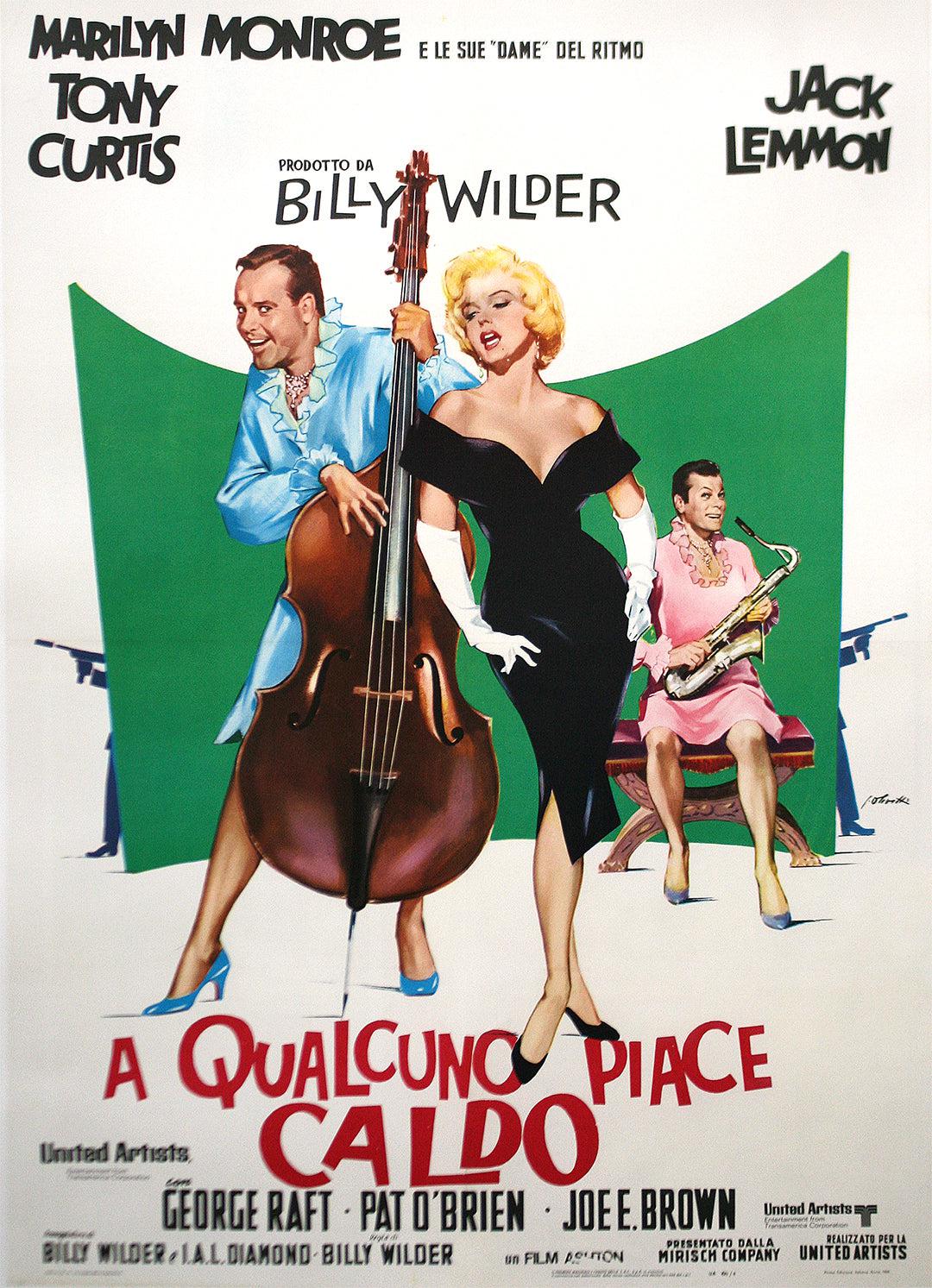This vintage movie poster for the film "Qualcuno Piace Caldo" prominently features a colorful, cartoonish illustration against a vivid green backdrop. At the top, the names of the stars appear in bold black letters: "Marilyn Monroe" followed by "Tony Curtis" and "Jack Lemmon". Just below, in white-on-black text, it reads "Prodotto da Billy Wilder," indicating the producer.

The central focus of the poster includes caricatures of the three main actors. Marilyn Monroe is depicted in the middle, radiating glamour in a low-cut black dress that emphasizes her iconic blonde hair and curvaceous figure. She accessorizes with elegant white gloves and classic black heels. 

To her right, Jack Lemmon is illustrated, humorously clad in a knee-length pink dress adorned with lacy white trim and matching high-heel shoes. He is sitting on a bench, engrossed in playing the saxophone with a cheerful expression. 

On the left, Tony Curtis is seen wearing a blue dress and blue high heels, holding and playing a cello with a smile, adding to the whimsical scene. The poster cleverly captures the comedic essence of the film with the male characters dressed in drag alongside the glamorous Monroe.

Additional cast members listed at the bottom include George Raft, Pat O'Brien, and Joe E. Brown, adding further depth to the ensemble. The film title "Qualcuno Piace Caldo" is displayed prominently in bold red letters at the bottom of the poster, amidst other production credits. The entire design conveys the vibrant, playful mood of the movie, drawing attention and sparking curiosity.